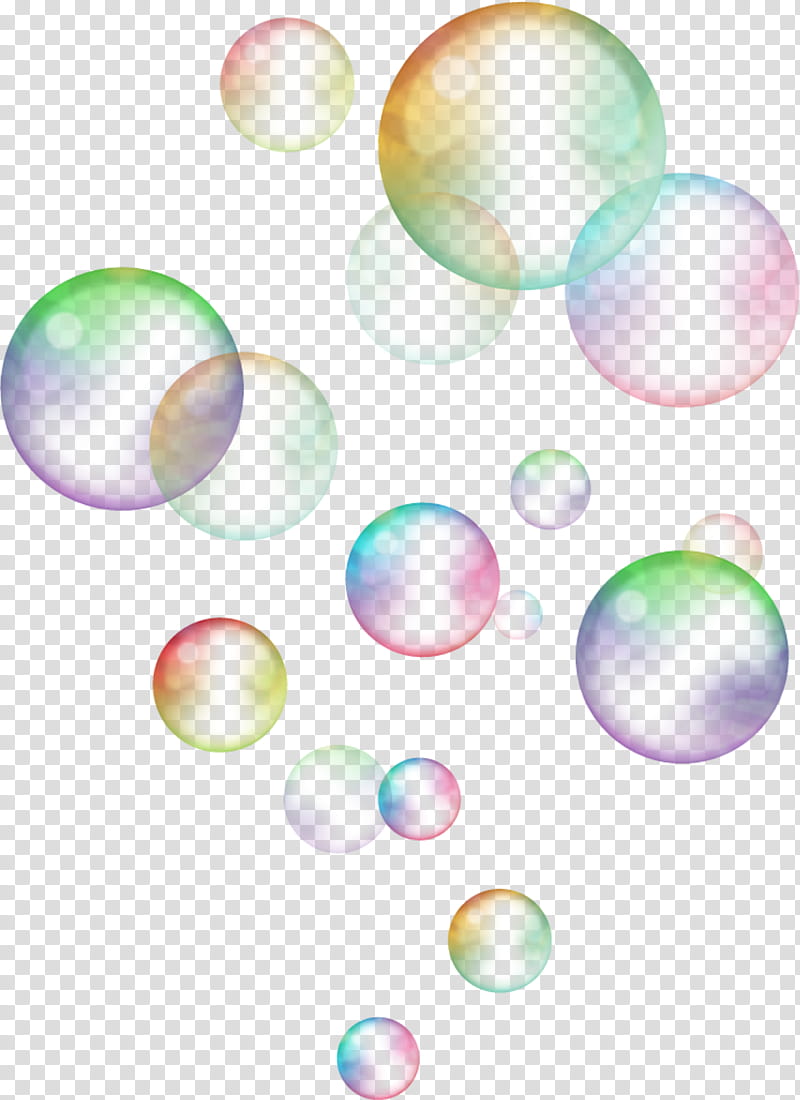This vertical rectangular image features a checkerboard background of alternating white and gray squares. Starting at the bottom, clusters of bubbles ascend towards the top, increasing in size as they rise. The largest bubble is slightly off-center to the right at the top of the image, though smaller bubbles are interspersed throughout the space above. Each bubble displays a mesmerizing gradient of colors, predominantly purple, green, orange, and yellow, with the colors radiating from the edges toward the center. The bubbles in the background appear more faded and less vibrant compared to the vivid bubbles in the foreground, creating a sense of depth and dimension throughout the image.